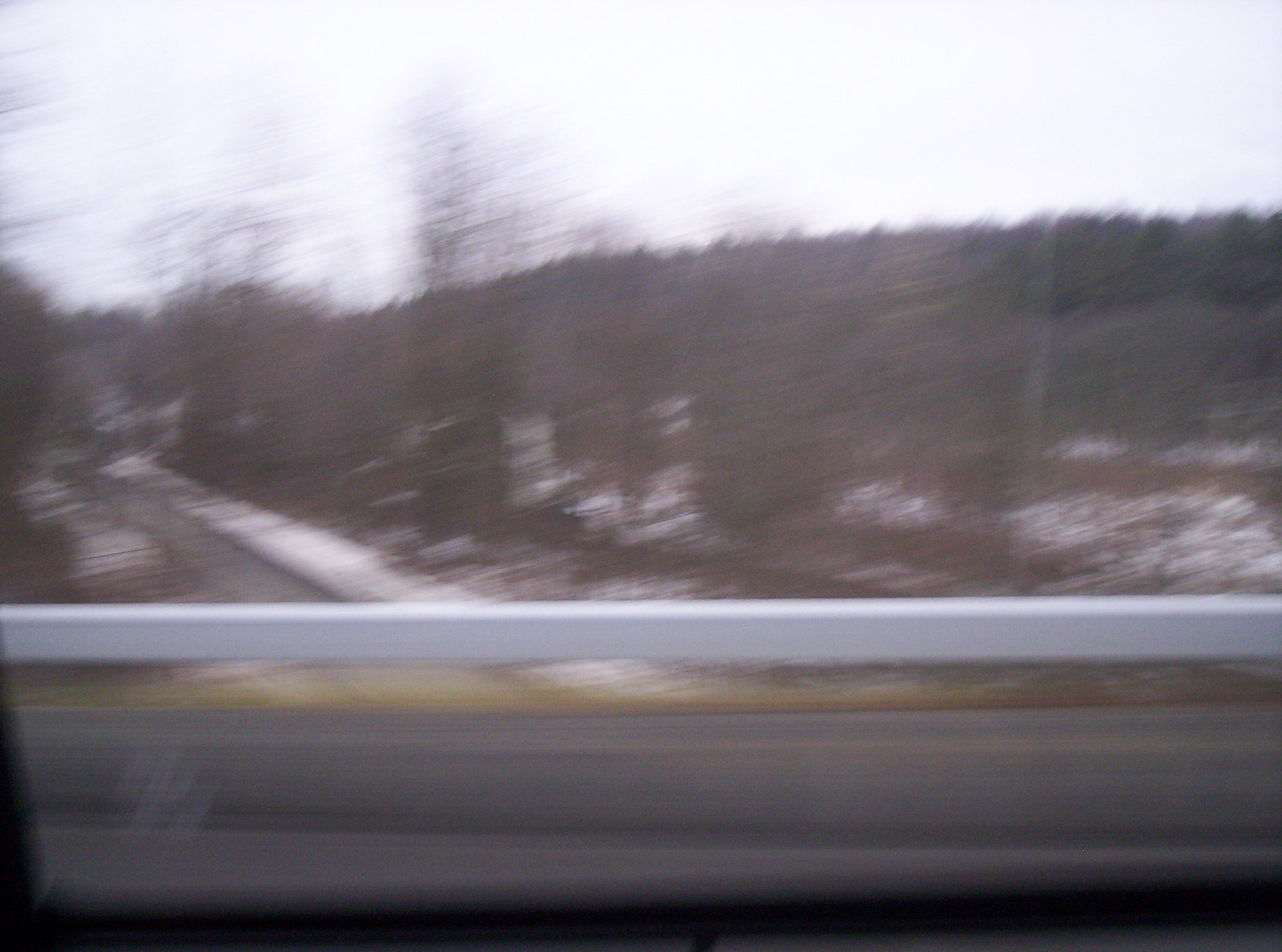The image is a point-of-view photograph taken from inside a moving car, capturing a scene along Edgemoor Road. The motion blur suggests the vehicle is driving fast, and the picture is slightly tilted downwards. The car’s doorframe and window glare are visible, along with a car label at the bottom left of the window. A long, white, metal-colored guardrail runs alongside the road, alongside a yellow road line and asphalt. Snow covers the ground, both on the roadside and up a hill in the background. The hill supports bare trees with no leaves, resembling those that grow in winter, with some looking like Christmas trees. The background reveals a mountainous area with brown grass and a valley below, possibly with train tracks, indicating the car is driving over a bridge.